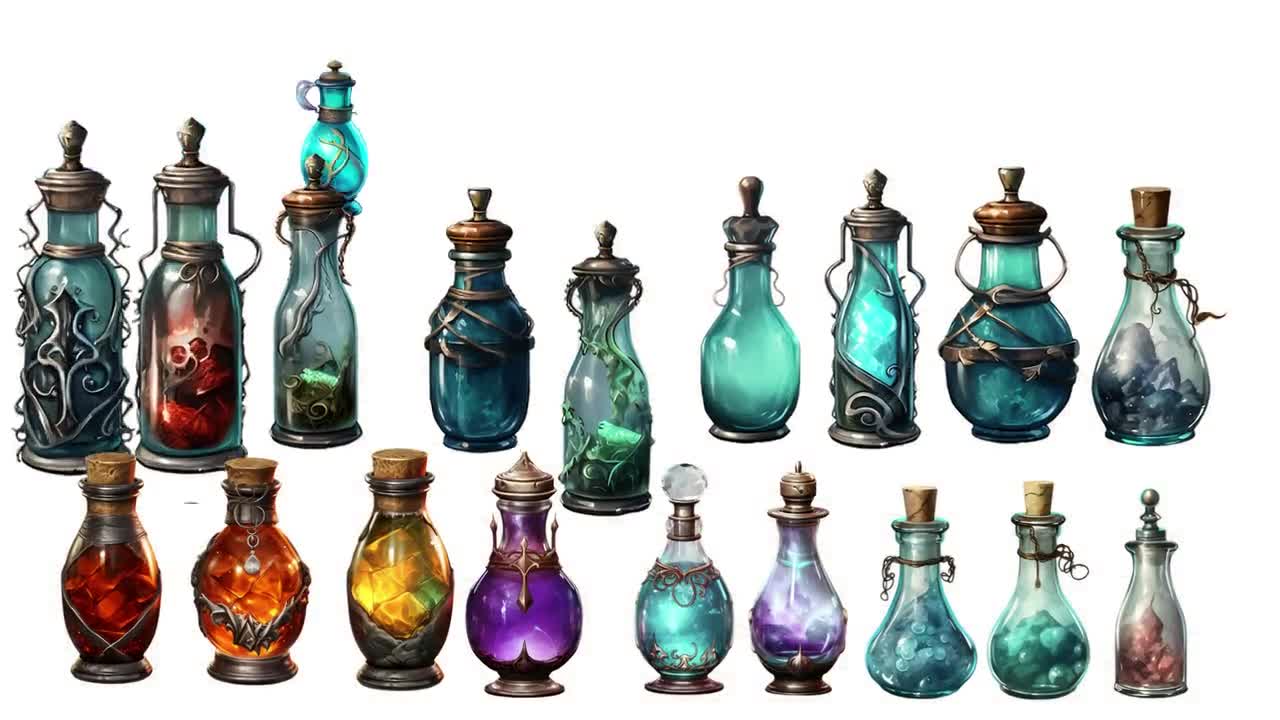This image features a collection of exquisitely crafted bottles, which appear to range in function from ornamental perfume bottles to potential cruets for oil. The bottles are predominantly clear but showcase a spectrum of hues from transparent to shades of gray, purple, and blue, possibly due to their varied contents. A striking yellow bottle stands out among them. Each bottle on the top row is adorned with ornate tops and intricate wire decorations encircling their bodies. Notably, the last bottle on this row is sealed with a cork. The bottom row largely consists of bottles with cork stoppers, and includes a remarkable crystal bulb bottle and two elegant silver ones. Each bottle seems to hold a unique substance, adding a layer of mystery and wonder to the collection.